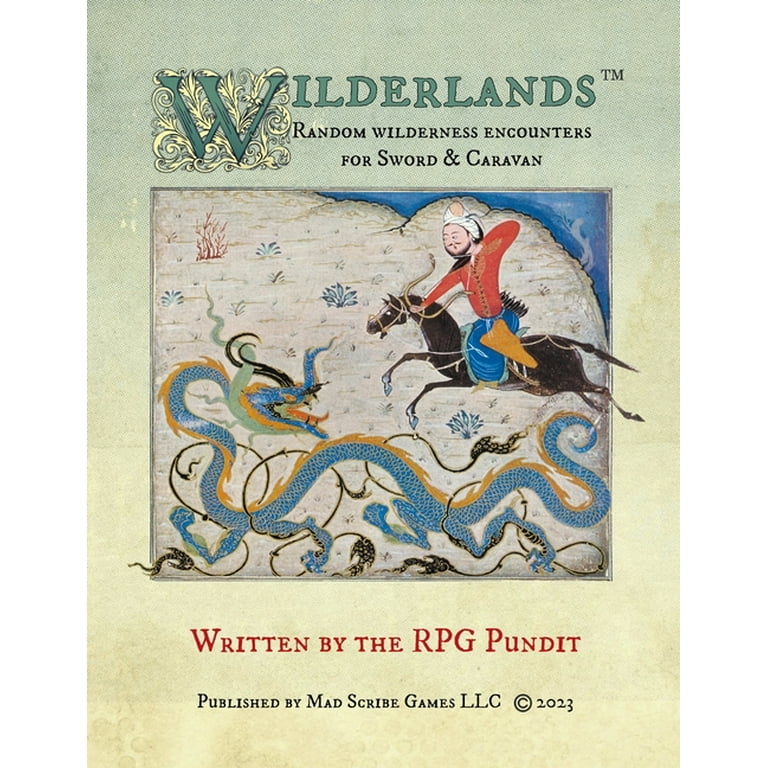The cover of the book "Wilderlands: Random Wilderness Encounters for Sword and Caravan," written by RPG Pundit and published by Mad Scryer Games LLC in 2023, features an enchanting and dynamic scene. Set against a light green background, the center of the cover illustrates a man wearing a white turban, red long-sleeved shirt, and blue pants or skirt, riding a dark brown horse with a bit of white on its front hooves. The horse appears to be in flight, magically soaring through the air. The man is depicted mid-action, shooting a bow and arrow towards a large blue dragon or sea serpent below him. The dragon, which stretches across most of the front, has four legs, gold scales on its back, and long black tendrils sprouting from various parts of its body. The book's title is written in green and black lettering at the top, while the author's name and publishing details are prominently displayed at the bottom in red and black letters.